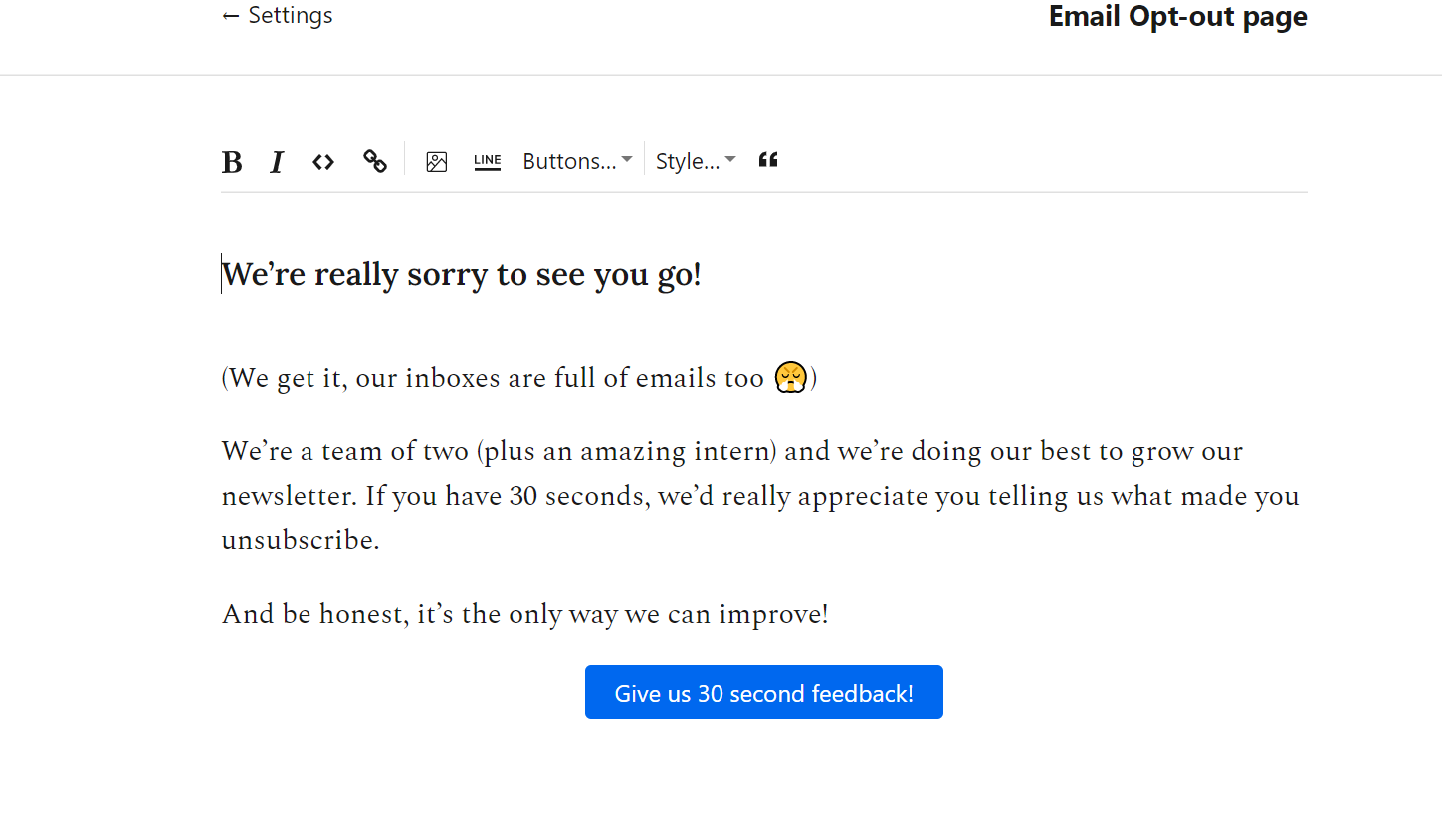The image depicts an email opt-out page in draft form, with a clean white background. The email's title is prominently bolded and reads, "We're really sorry to see you go!" Below this title, the body of the email starts with a parenthetical aside, "(We get it, our inboxes are full of emails too)," accompanied by an exhausted, irritated emoji. The following message reads, "We're a team of two (plus an amazing intern) and we're doing our best to grow our newsletter. If you have 30 seconds, we'd really appreciate you telling us what made you unsubscribe. And be honest, it's the only way we can improve!" An exclamation point punctuates the sentence for emphasis.

Beneath the text, there is a blue button with white font, inviting the user to "Give 30-Second Feedback" regarding the unsubscribe decision. The email draft appears to be incomplete and has not yet been sent.